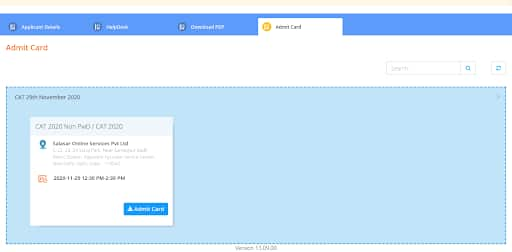The image portrays a web page displayed in a landscape orientation. The topmost section features a thin, pale orange bar with no text. Below this is a gap, followed by a navigation bar in a light blue hue containing four tabs or links. Three of the tabs are on the blue background, but the fourth tab is highlighted in white, indicating it has been selected. This highlighted tab reads "Admit Card" in black font, accompanied by an orange icon to its left.

Directly below this bar, another row displays the text "Admit Card" in bold orange font, with a search bar situated on the right side of this section. Beneath this, on a light blue background, appears the designation "CAT" in uppercase letters followed by "29th of November 2020" in lowercase, all in black font.

Additionally, within this pale blue segment is a white rectangle containing various pieces of information. It prominently displays "CAT 2020" in capital letters, followed by "non-PWD/cat 2020." This section also includes some other details not specified in the caption and features a clickable button labeled "Admit Card" in white font on a blue background, with a white triangle icon to the left of the text.